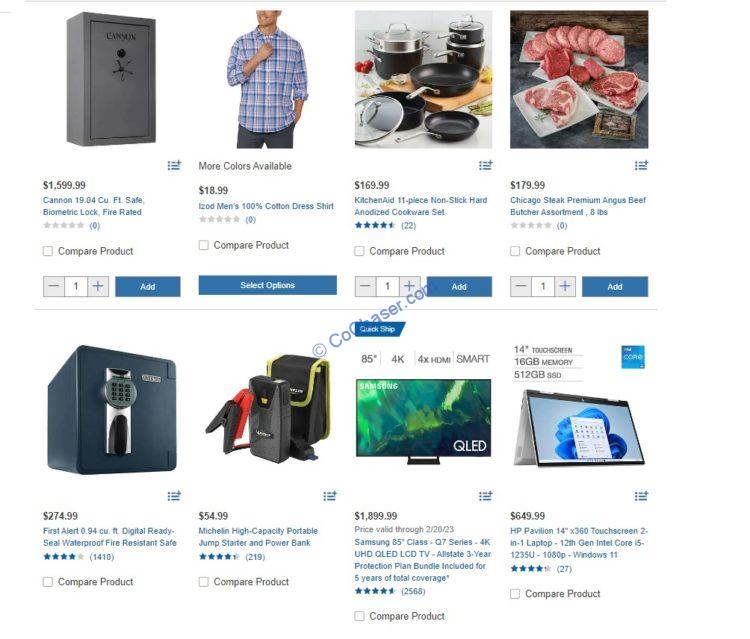Here is the cleaned-up and detailed descriptive caption for the image:

---

The image depicts a retailer's online product listing page with several items on display, each presented against a white background. Each product includes a photograph, title, description, and price. For example, located in the top left corner is a **Canon 19 Cubic Feet Biometric Safe**, fire-rated and featuring a black exterior with "Canon" printed on the door. This item is priced at $1,599.99 and has a blue "Add" button below it.

Next to this is a **Men's Flannel Cotton Dress Shirt**, priced at $18.99. Below this item, there are options to compare the product and select different options, along with a blue button for selection. 

Overlaying the center of the webpage is a watermark reading "copyrightcoachaser.com," indicating a copyright notice.

On the bottom right of the second row is an **HP Pavilion 14-inch 360 Touchscreen 2-in-1 Laptop**. This device features a 12th generation Intel Core i5 processor and runs on Windows 11. It is shown with a rating of four stars based on 27 reviews. The product image displays an Intel Core logo in the top right corner. Additionally, the top left of this product description highlights key specifications: "14-inch touchscreen, 16GB memory, and 512GB SSD."

---

This caption provides a detailed and organized description of the retailer's product listing page, highlighting specific products and their attributes.